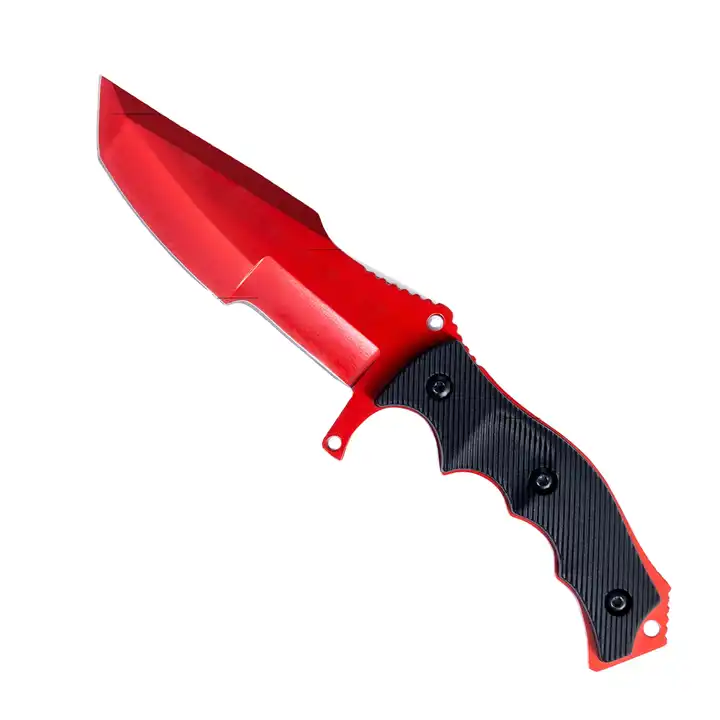This detailed close-up image features a gleaming, new pocket knife set against a white background. The knife's blade is a striking bright red, measuring approximately five to six inches in length, extending to the top-left corner of the image, with a sharply pointed tip. The blade itself is smooth aside from a section of ridged notches near the handle.

The handle, oriented towards the bottom-right, is black with diagonal lines providing a textured grip. This black section is secured to the red metal handle plate with three black phillips head screws, visible at the top, middle, and bottom of the handle. Additional details include a circular hole at the bottom and two holes near the base of the blade, all in the red portion of the handle.

Overall, this pocket knife presents a modern and functional design, with a polished, sharp blade and a meticulously designed handle for optimal grip and control.